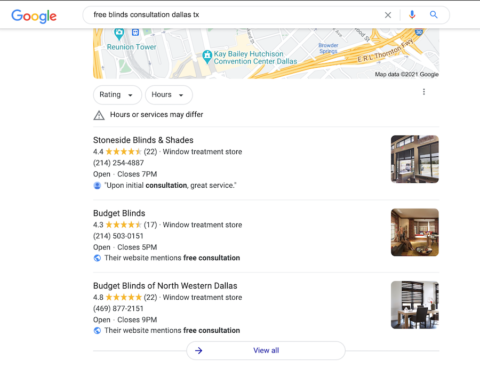This image is a screenshot of a Google search results page, primarily focused on window treatment companies. At the top of the screenshot is a light gray horizontal line, beneath which lies a white rectangle spanning horizontally. Inside this white area, on the left, the "Google" logo is displayed in its characteristic multicolors. To its right is a search bar, which includes features such as a cancel button (X), a microphone icon for voice search, and a magnifying glass symbolizing the search action.

Below this search bar, the page transitions into a split display: the lower half reveals a segment of a Google Map, and further down are search results listing three companies. Each listing includes comprehensive details: the company name, a star rating indicative of user reviews, a phone number for immediate contact, and the operational hours.

The three companies featured are:

1. **Stone Side Blinds and Shades**
2. **Budget Blinds**
3. **Budget Blinds of Northwestern Dallas**

To the right of each listing, there is a square photograph showcasing the exterior of each respective company's building, providing a visual point of reference.

At the very bottom center of the screenshot, there's a horizontally elongated oval button. On the left side of this button is a blue right-pointing arrow, while the center of the button is inscribed with "View all" in blue text, indicating an option to see more search results.